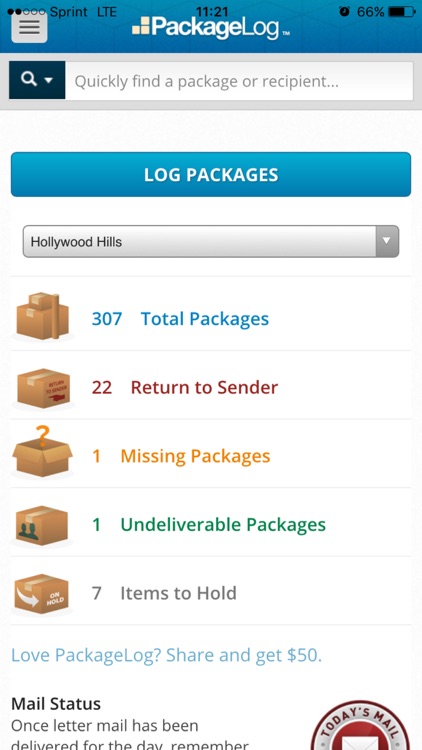A vertical portrait screenshot taken on a smartphone, displaying an app interface called "Package Log". At the top of the screen, the phone's status bar shows a Sprint LTE service indicator, the time as 11:21, an alarm icon, and a battery level at 66%. 

Below the status bar, there is a search bar with a search button to its left. Further down, a large button labeled "Log Packages" is prominently displayed. Under this button, a drop-down menu indicates the location "Hollywood Hill" is selected.

The screenshot details several package statuses in a list format: 
- 307 total packages
- 22 returned to sender
- 1 missing package
- 1 undeliverable package
- 7 items to hold

Below these indicators, there is promotional text stating "Love Package Log, share and get $50". Additionally, the mail status is summarized as "One letter of mail has been delivered for the day" with a reminder below it. To the right, there is an emblem labeled "Today's Mail".

The interface is slightly cut off at the bottom, omitting the minimize, back, and applications buttons typically found on the phone's navigation bar.